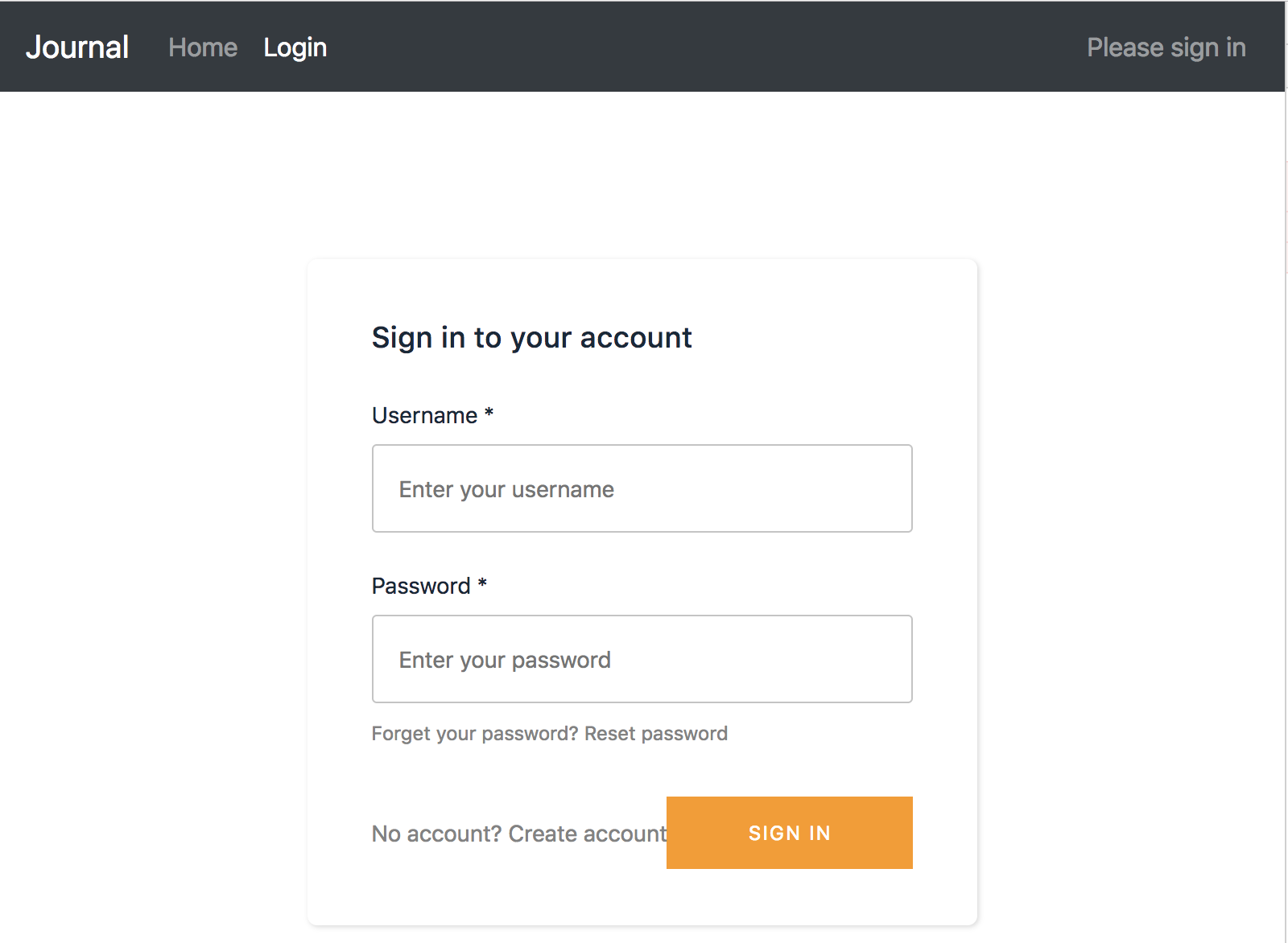This image depicts the sign-in page for a website named "Journal." The website's name, "Journal," is prominently displayed in the upper left-hand corner inside a black rectangle that extends across the width of the page. Adjacent to the site name are two navigation options: a home button that takes you to the homepage, and a login button for user access. 

On the right-hand side of this black rectangle, the page provides status updates related to the sign-in process, stating "Please sign in" to prompt users to log in before gaining further access.

Below this header is the main sign-in area, which is a typical rectangular box familiar to most internet users. At the top, the text "Sign in to your account" is displayed in dark black font. The sign-in form consists of two fields: the first field, labeled "Enter your username," allows users to input their username, and the second field, labeled "Enter your password," is for the user's password. Both fields are rectangular text boxes.

Below the password field, there are options for users who have forgotten their username or password, providing information on how to address such issues. Finally, at the bottom of the sign-in area is a bright orange button with small white text that reads "Sign in," inviting users to complete the login process.